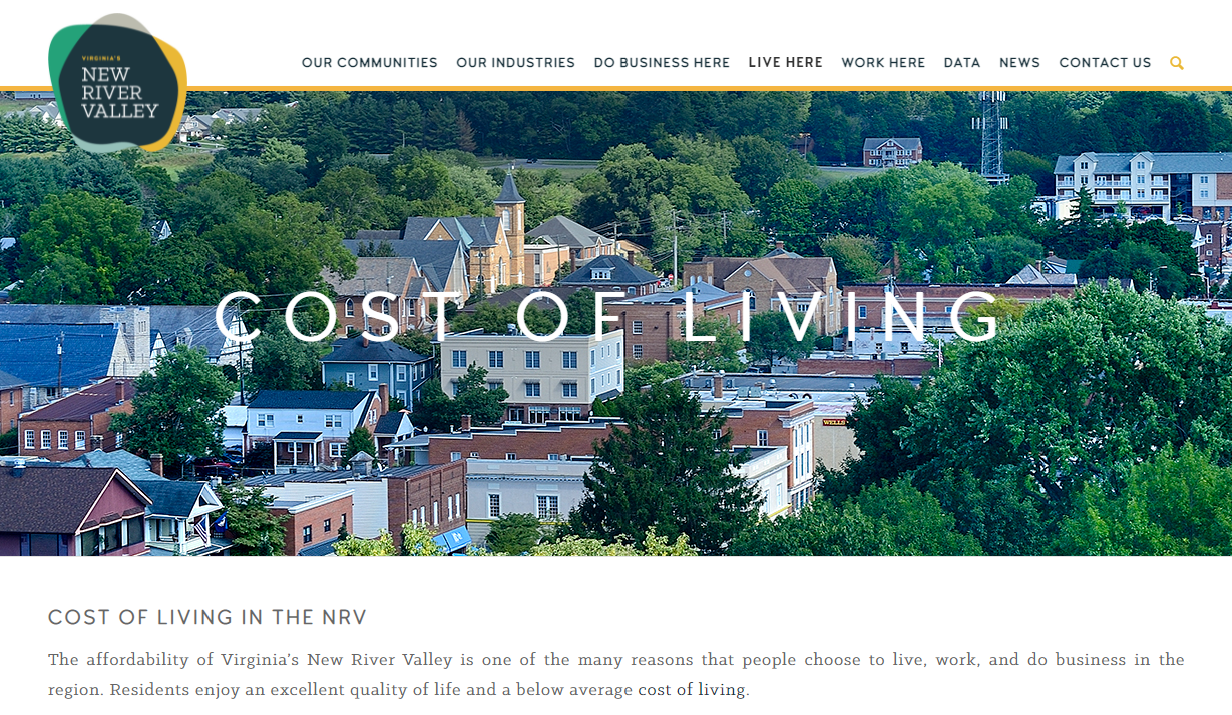This screenshot captures the homepage of the New River Valley website. In the upper left corner, a black section prominently features the white text "New River Valley," encircled by segments in various colors forming a flower-like shape: green on the upper left, purple at the top, yellow on the right, and blue at the bottom. 

Across the top of the page, a navigation menu displays options in black text on a white background: Our Communities, Our Industries, Do Business Here, Live Here, Work Here, Data, News, and Contact Us. To the right, a yellow search icon is also visible.

The main image showcases a picturesque community characterized by numerous brick buildings, including a notable brick church. The scene is dotted with white buildings and abundant green trees, with an antenna visible in the background on the upper right. Overlayed on this image are large white letters that read, "Cost of Living."

At the bottom of the screen, a white section reiterates the "Cost of Living in the NRV" message and adds a description: "The affordability of Virginia's New River Valley is one of the many reasons that people choose to live, work, and do business in the region. Residents enjoy an excellent quality of life and a below-average cost of living."